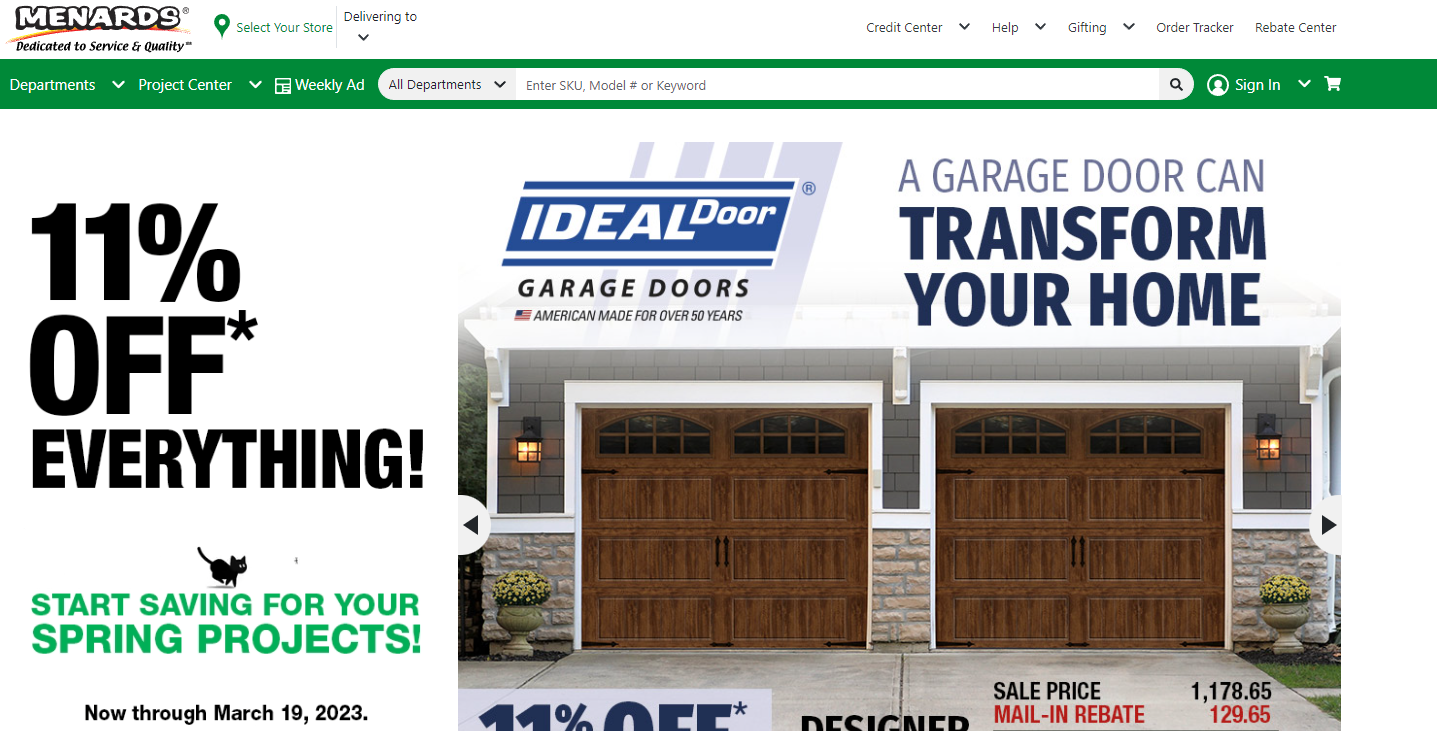This detailed caption describes an advertisement image from Menards, a hardware store, featuring a promotion on garage doors:

In this promotional image from Menards, the hardware store is showcasing a sale on garage doors. The image prominently displays a large banner with "11% Off Everything" written in bold black letters. The advertisement highlights "Ideal Garage Doors - American Made for Over 50 Years," emphasizing the quality and longevity of the product. The main feature of the image is a photograph of two brown paneled garage doors installed on a stylish house with a stone facade halfway up, complementing the brown exterior. The ad copy states, "A garage door can transform your home," and encourages customers to "Start Saving for Your Spring Projects." Notably, the sale runs through March 19th, 2023, as indicated by the text at the bottom. In addition to the large discount, the image mentions a specific sale price of $1178.65 with a mail-in rebate of $129.65. The search bar at the top reads "Enter SKU, model number, or keyword," over a green section, which includes navigation links for "Departments," "Project Center," and "Weekly Ad." The image is topped with a whimsical touch—a picture of a black cat running. The overall layout suggests a push for seasonal savings on home improvement essentials.